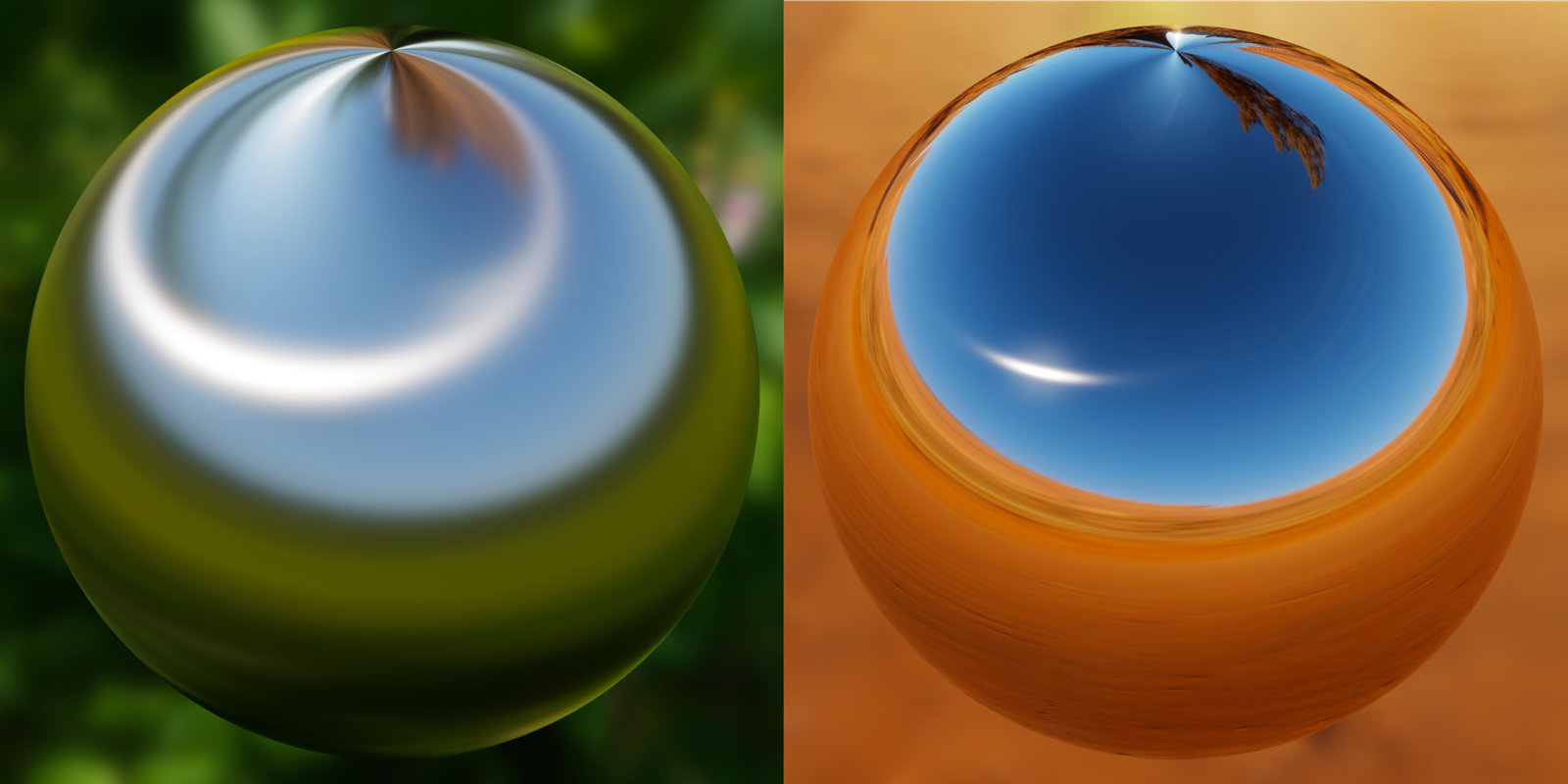The image is divided into two sections, each showcasing a meticulously photographed metal sphere. On the left-hand side, the sphere appears smooth and gray, set against a green background that suggests out-of-focus plant life. This sphere reflects a clear blue sky, verdant greenery, and a dominant ring of white. On the right, the metal sphere has a backdrop that is a blend of orange and brown, evocative of desert sand, although it is also out of focus. The sphere mirrors this sandy environment, coupled with a hint of a blue sky overhead and the blurred reflection of a brown tree at the top. Both spheres are central, brilliantly coordinated, and evoke a sense of artistry with their vivid and contrasting color palettes — greens, blues, oranges, and browns — and their reflective surfaces that capture their respective backgrounds with a painterly, almost surreal quality.